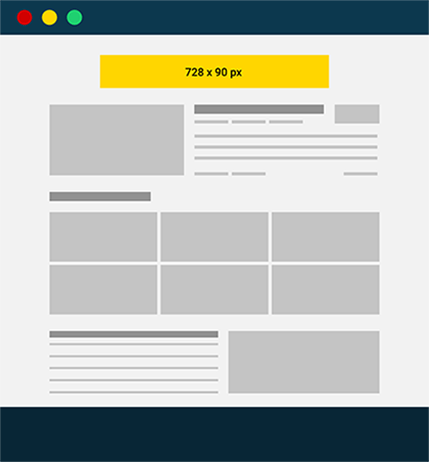This image displays a template designed for a news or information website, complete with designated sections for text and images. The layout is framed by two long, rectangular, bluish-black boxes at the top and bottom. At the top border, there are three sequentially placed colored circles: red, yellow, and green. 

Below this, the template mimics the format of a newspaper page, providing structured placeholders for content. Prominently featured is a yellow rectangular box with bold black text that reads "728 x 90 PX," suggesting an advertisement space.

The main body of the template includes eight rectangular placeholders for images, which could also serve as spots for a logo. There are two to three text placeholders distributed throughout, ideal for titles or descriptive text. The lighter gray boxes indicate where images could be placed, while darker gray lines suggest the format for headings or captions. The template is versatile and does not specify usage for web pages, computers, or smartphones, focusing instead on the layout structure itself.